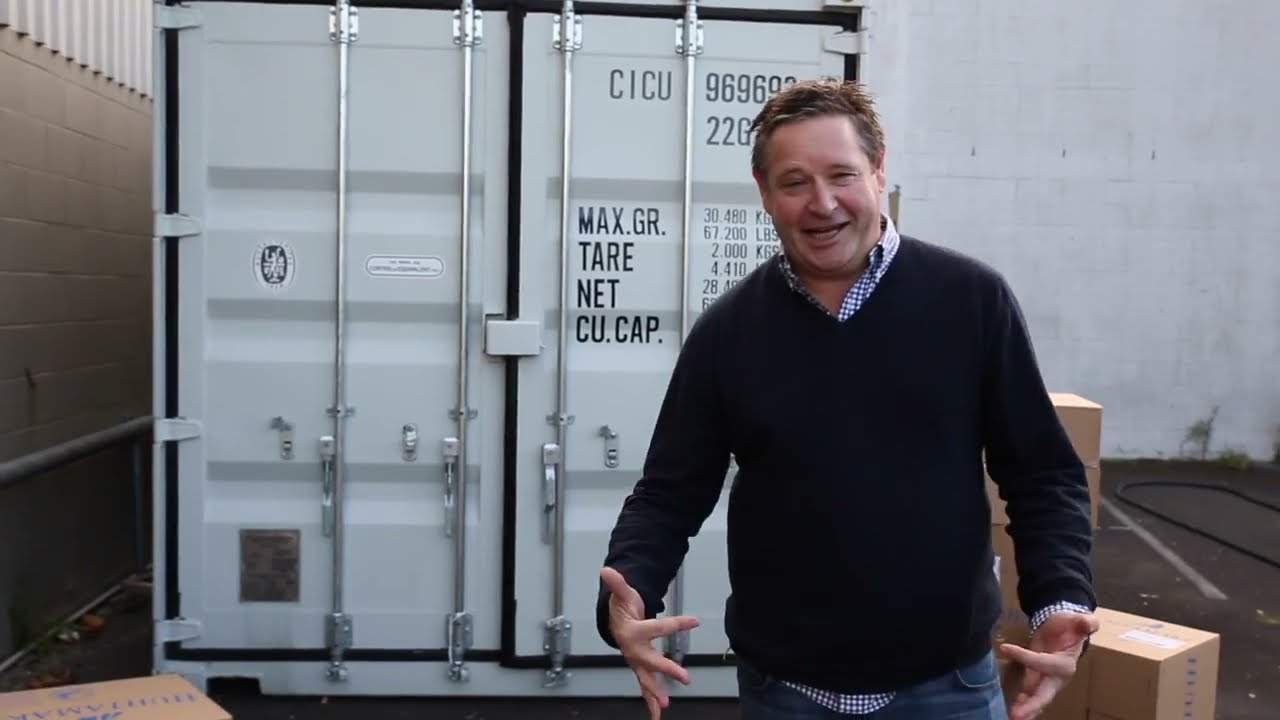The photograph features a chubby white man with short, spiked black hair tinged with gray at the temples, standing in the center of the image in front of a building. He is squinting, possibly appearing a bit hungover. The man is dressed in a navy blue sweater over a blue and white checkered collared shirt. He stands before a rectangular white-framed sign with a red background that has partially obscured text, only revealing the word "door." Behind him, the building's façade shows a lower section of deep brown color and an upper section filled with numerous windows, each bordered by black metal lining and adorned with white curtains. In the bottom right corner of the image, there is a white asterisk followed by the word "Hastings" in large white text.